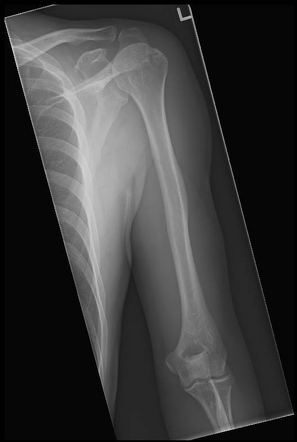The image is a highly detailed x-ray photograph showcasing a section of a human body. The x-ray is positioned diagonally from the top left corner to the bottom right corner, set against a solid black background. It primarily captures a portion of the torso, specifically the left shoulder extending down to just past the elbow. Clearly visible within the image are the ribcage on the left, the shoulder joint, and the arm bones all the way to a blurred depiction of the hand. The x-ray exhibits varying shades of gray, with highlights in white and black, and it is formatted in a rectangular shape. The image suggests a possible fracture or dislocation near the shoulder, indicative of the thin and slightly muscular frame captured. Notably, the x-ray includes the marking "L" at the upper part of the picture, likely designating the left shoulder. The overall setting and style of the imagery are consistent with standard medical radiography.